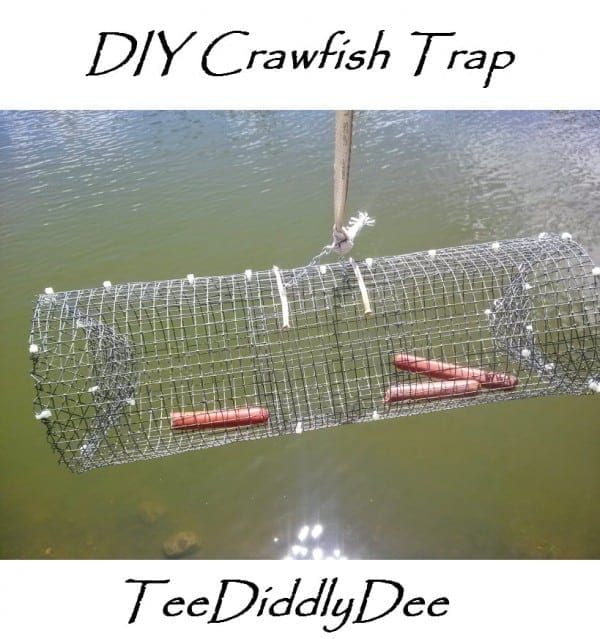This detailed image appears on a blog and showcases a DIY crawfish trap. At the top of the image, “D.I.Y. Crawfish Trap” is prominently displayed in black letters, clearly indicating the purpose of the trap. At the bottom of the image, a watermark or credit reads “T. Diddley D.” The trap itself, held aloft over what seems to be a pond or lake with murky, army-green water, is a rounded, cage-like structure made from chicken wire. It features a narrow cone on both ends to prevent crawfish from escaping once they enter. The trap is held together with plastic zip ties or wire ties, and has a strap attached for lowering and lifting it. Inside the trap, three hot dogs serve as bait, enhancing its DIY, homemade feel. The reflection of light on the water's surface adds a natural touch to the setting.